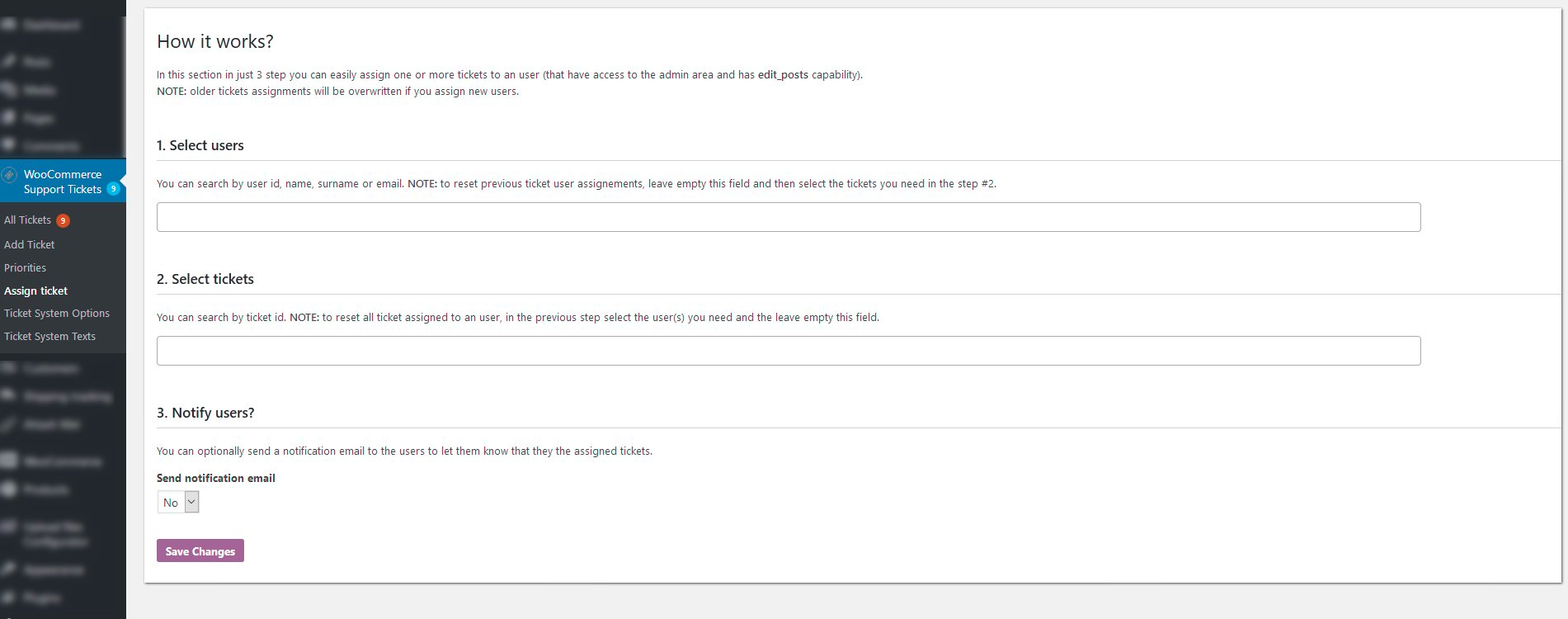The image shows a cropped screenshot of a ticket sales website, specifically highlighting the "Support Tickets" tab. On the left side of the interface, there are several menu options such as "All Tickets," "Add Ticket," "Priorities," "Assign Ticket," "Ticket System Options," and "Ticket System Tools." The purpose of this section is ticket management, presumably for customer support or internal task tracking, rather than for aviation or airplane ticket sales.

On the right side, a detailed three-step guide explains the process of assigning tickets to users:

1. **Select Users**: A text description is provided, though it is too small to read clearly. An empty text bar allows for the entry of user information.
2. **Select Tickets**: Again, accompanied by a small, unclear text description and another bar for selecting specific tickets.
3. **Notify Users**: This section is legible and explains that you can notify users via email regarding their assigned tickets. Options include a dropdown menu to choose whether to send a notification email, followed by a purple "Save Changes" button to confirm updates.

The interface appears to be intuitive, consolidating ticket management features for administrators with editing capabilities.